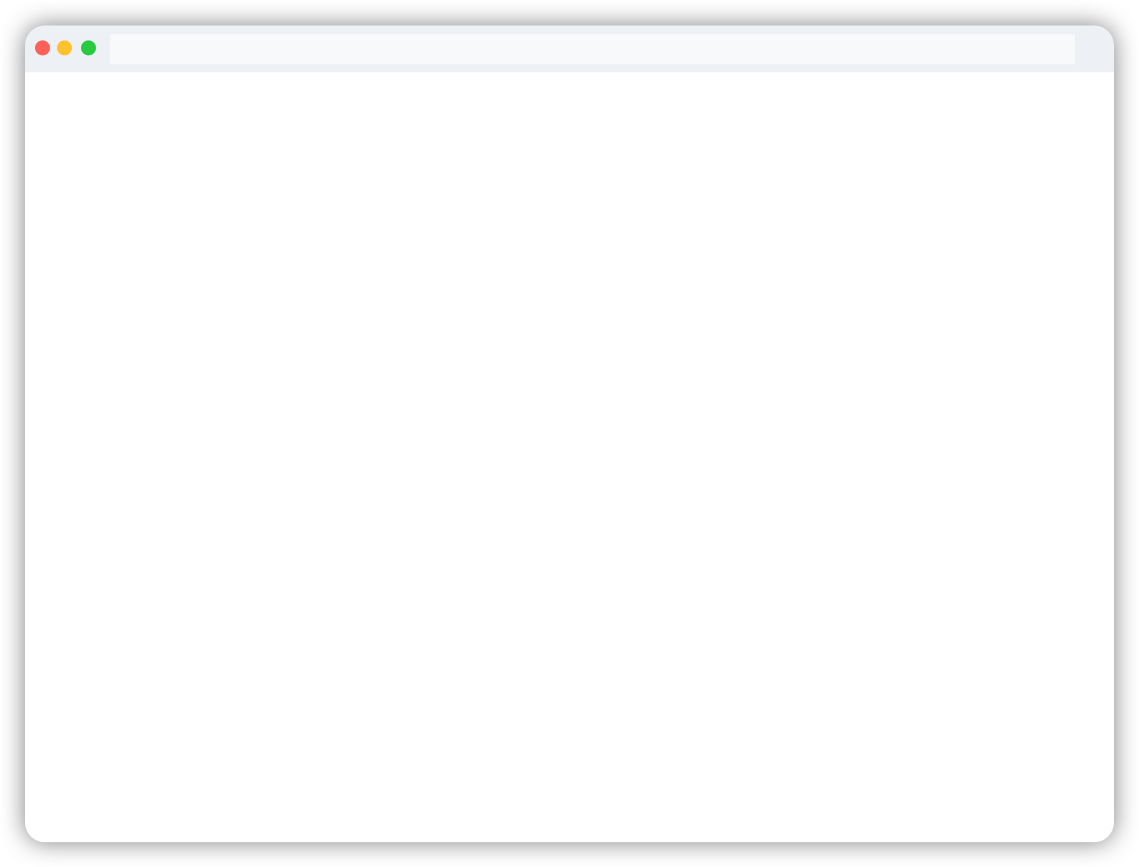The image is a stylized representation of a web browser window rather than an actual screenshot. The overall shape of the browser is a square with subtle, light gray borders that exhibit a slight gradient to create a shadow effect, adding a sense of depth. Notably, the corners of this square are softly rounded, enhancing the clean, modern aesthetic.

At the very top of the browser window, there is a horizontal border that spans almost the entire width. This border is also very light gray, contributing to the cohesive minimalistic design. Positioned within this top border is a white address bar, which, in a real browser, would display the website URL; however, it is blank in this depiction.

On the upper left corner of the browser window, there are three small, circular buttons aligned horizontally. The leftmost circle is red, the middle one is yellow, and the rightmost one is green, mimicking the window control buttons commonly found on macOS interfaces.

The central portion of the browser window, which would typically display the web page content, is completely blank, represented by a white, empty space. This blank white page emphasizes the simplicity and straightforwardness of the overall design. The entire composition captures the essence of a web browser interface in an elegantly minimalistic manner.